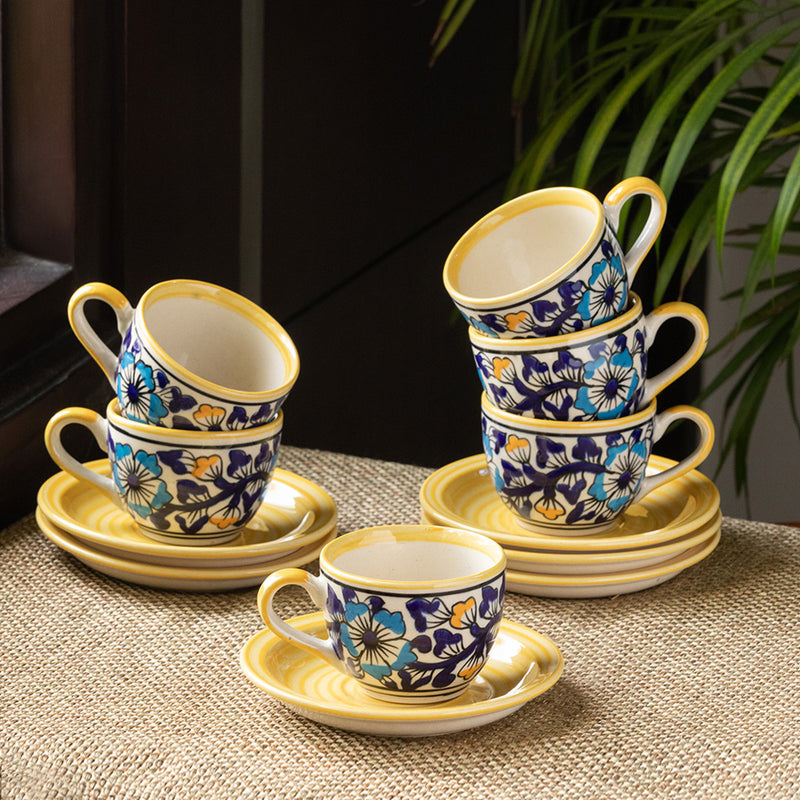In the color photograph, various teacups and matching saucers are artfully arranged on a table covered with a light brown linen tablecloth. At the center of the composition, a single cup is perched on a yellow saucer with white on the bottom. The cup showcases a white background adorned with a floral design featuring orange, purple, and turquoise-accented flowers, along with a yellow rim and handle.

To the left, a stack of two saucers supports two cups, both bearing the same floral pattern and yellow accents as the central cup. On the right, three teacups are precariously stacked on three saucers, with the top cup leaning slightly towards the middle. Each of these saucers also displays yellow concentric circles, adding a glossy, light yellow hue to the visual.

In the background, lush green leaves peek from what appears to be a palm tree, adding a natural contrast to the structured arrangement of the tableware. The room itself features wooden structural elements that frame the scene, complementing the ceramic aesthetic of the cups and saucers.